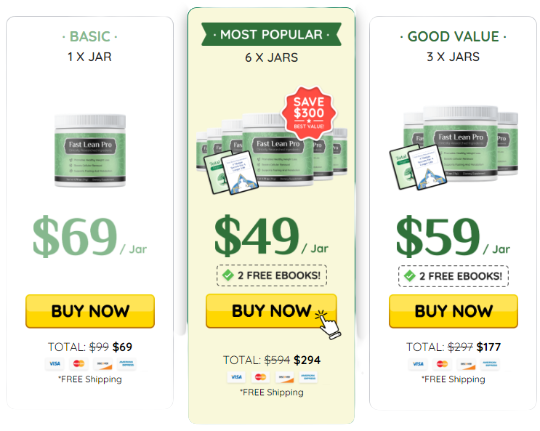The image is a three-panel graphic showcasing different purchasing options for Fast Lean Pro, emphasizing savings with larger quantities. 

- **Left Panel:**
  The basic option features a single jar priced at $69. The jar is cylindrical with a wide mouth, a white cap, and a green label. A black rectangle prominently displays "Fast Lean Pro" in white text, with three rows of smaller, illegible black text underneath. 

- **Center Panel:**
  Highlighted as the most popular choice among customers, this option offers six jars. Each jar costs $49, saving customers $300 in total. Additionally, this purchase includes two free eBooks. 

- **Right Panel:**
  The good value option offers three jars at $59 each. This deal also comes with two free eBooks. 

Beneath each panel, there is a yellow "Buy Now" button with black text, inviting customers to make a purchase.